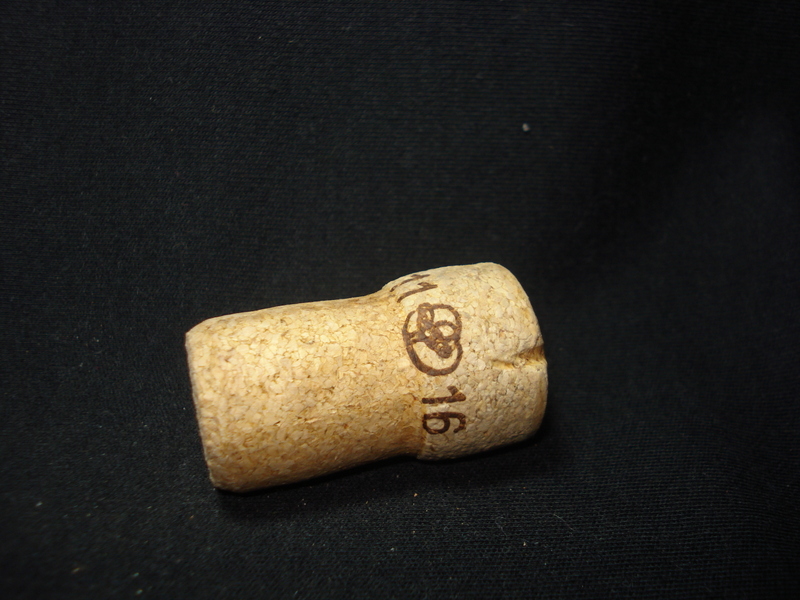This detailed photograph captures a champagne cork positioned on a piece of black felt fabric. The image, taken from above, prominently displays the classic mushroom shape of the light brown cork, indicating its probable cork and plastic composition. The cork features several distinct markings: on the left side of the top portion, the number "11" is printed in dark brown. Adjacent to this, in the center, is a small emblem resembling a circle with either a bumblebee or a simple tree in the middle. To the right of this emblem is the number "16." The top of the cork also shows a subtle groove, suggesting its purpose for securing the cork in place. These details stand out clearly against the minimalist black background, emphasizing the cork's intricate design and texture.